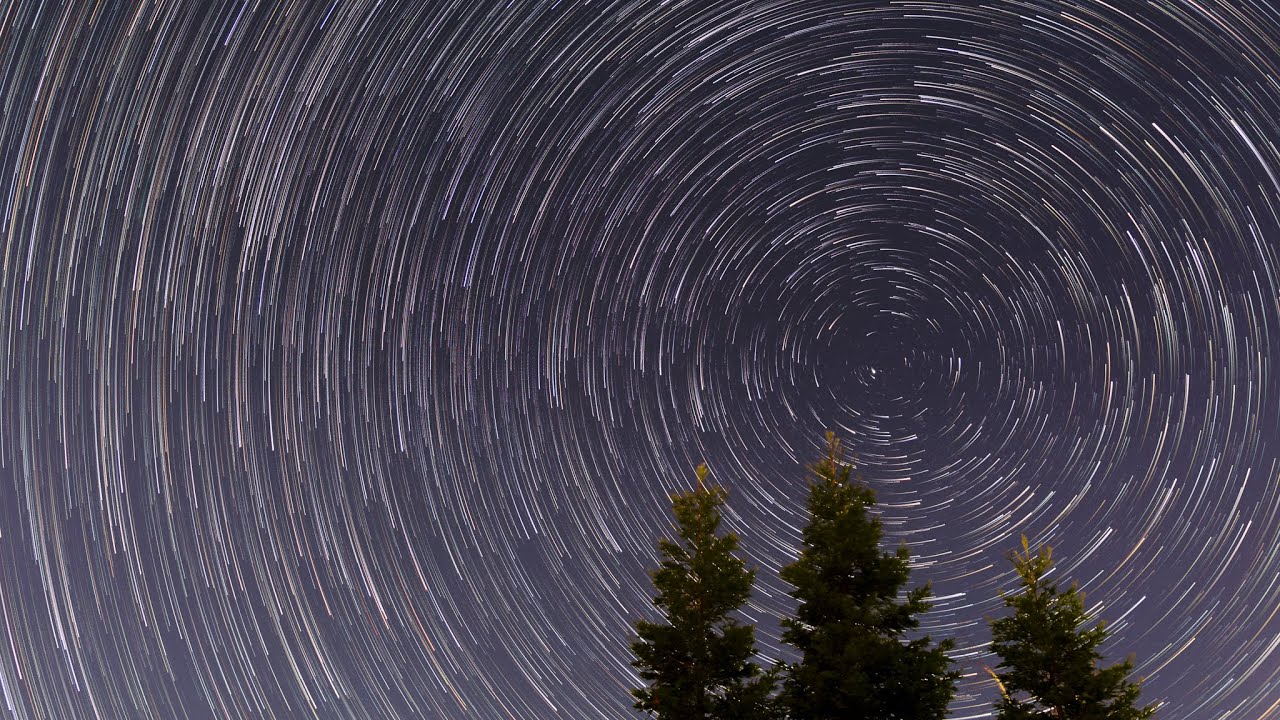The image is a complex and intriguing composition featuring three green-topped pine trees emerging from the bottom left-hand corner. The tops of these trees, stark against the darker background, appear shadowed and detailed. Dominating the scene is a dark gray, almost blue-gray sky filled with intricate white spiral patterns that converge towards a central point, creating a mesmerizing circle effect reminiscent of a long-exposure photograph capturing star trails or the swirling motion of a vortex. The meticulously crafted white lines create a sense of continuous motion, adding depth and dynamism to the dark and moody backdrop. The overall scene is both mysterious and surreal, leaving viewers to ponder its authenticity and the technique behind its creation.